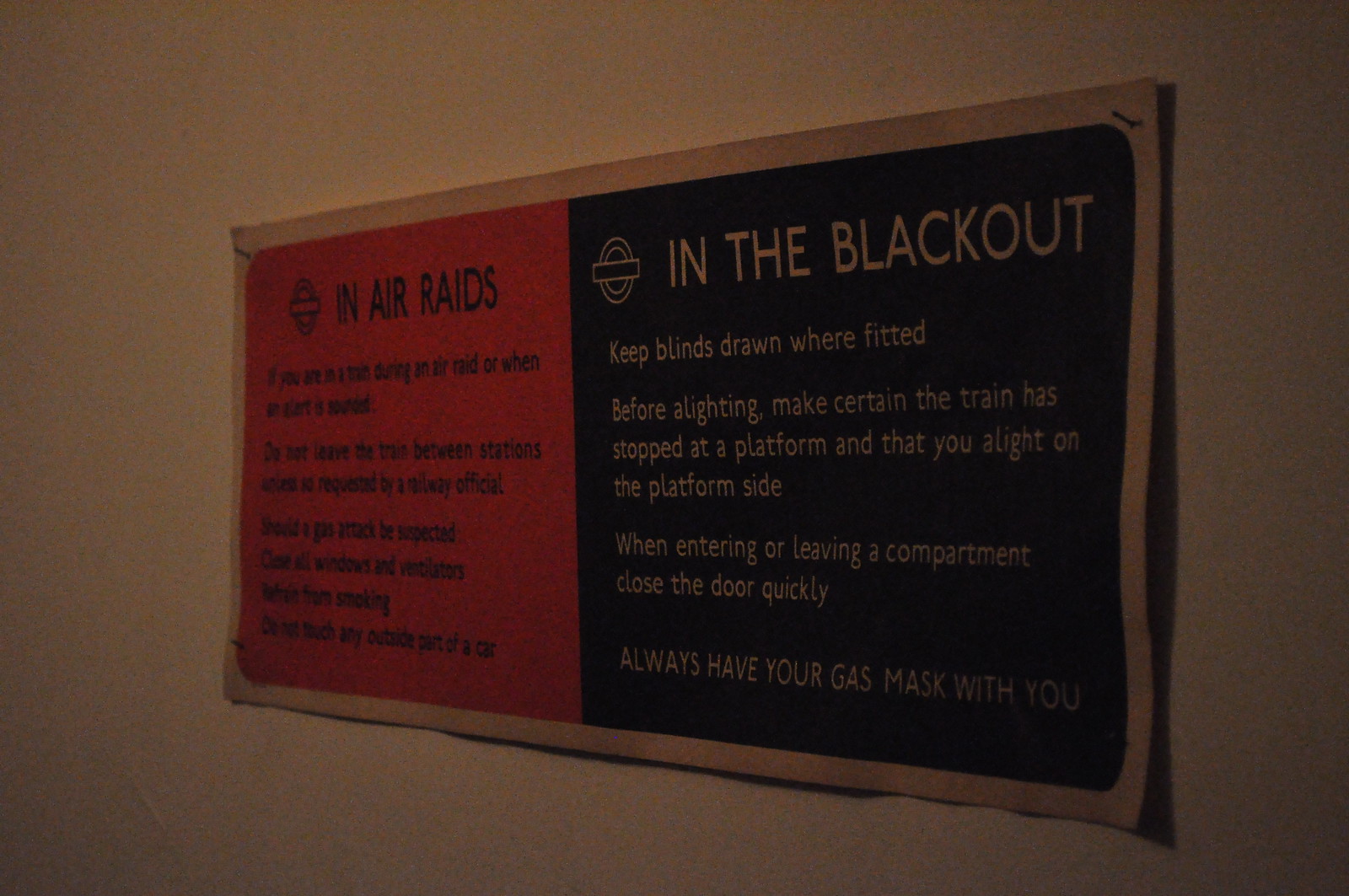The photo depicts a vintage World War II-era sign affixed to a tan wall with staples. The room appears quite dark, amplifying the sign's stark instructions. The sign itself is divided into two sections: the left side features a red background with black text, while the right side displays a black background with white text. 

On the left side, the header "In Air Raids" is prominent. This section contains critical instructions for train passengers during air raids: "If you are in a train during an air raid or when an alert is sounded, do not leave the train between stations unless requested by a railway official. Should a gas attack be suspected, close all windows and ventilators. Refrain from smoking and do not touch any outside part of a car." 

The right side, titled "In the Blackout," advises passengers to keep blinds drawn before alighting. It further instructs them to ensure the train has stopped at a platform, and to alight or enter only on the platform side. Passengers are also reminded to close the door quickly upon entering or exiting and to always carry their gas masks.

The sign is bordered in brown, adding to its vintage appearance, and provides a glimpse into the precautionary measures suggested during wartime train travel.